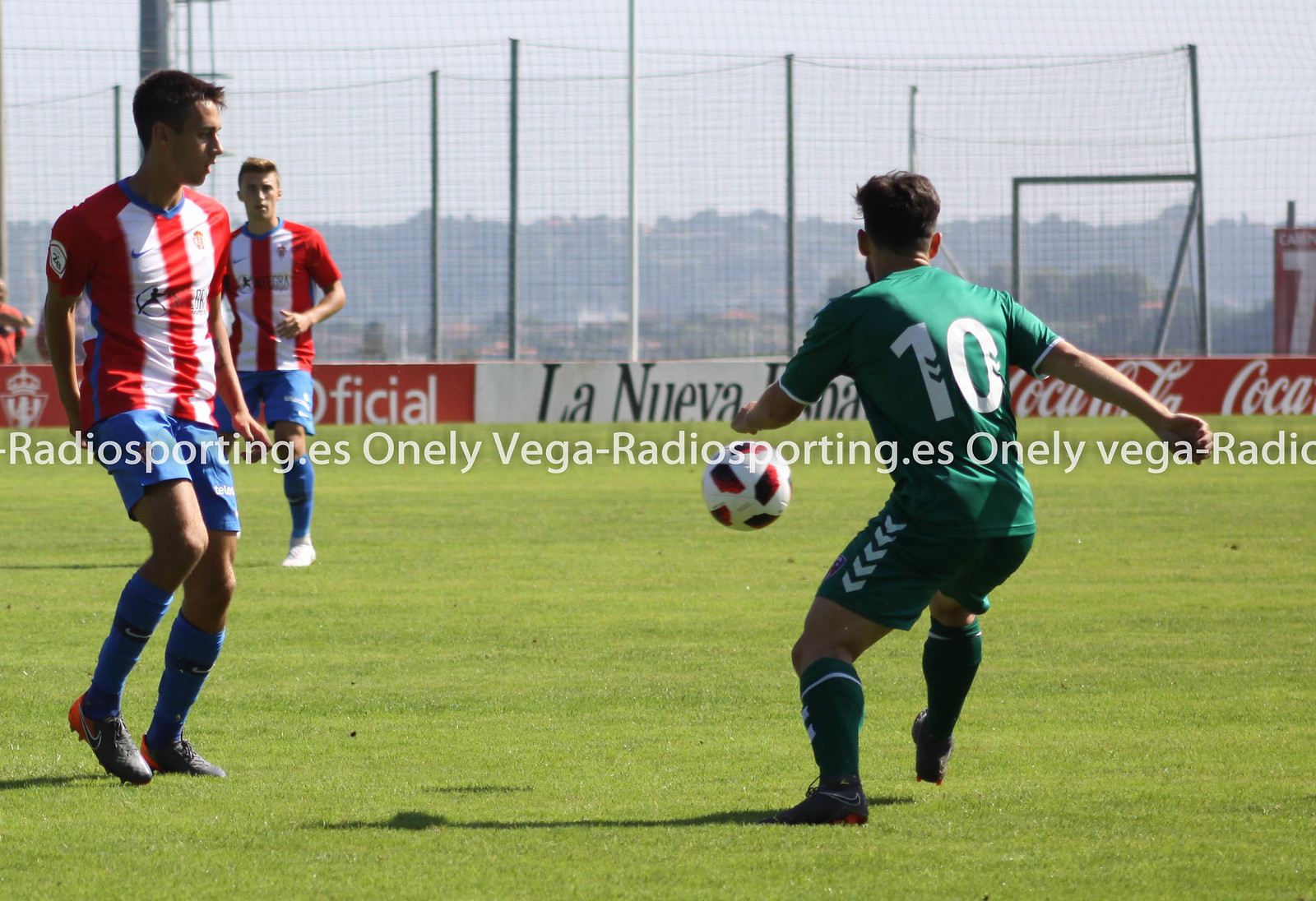In this horizontally aligned rectangular image, three soccer players are depicted on a lush green grass field. The player on the right, geared in a green and white uniform with the number 10 emblazoned in white on his back, is captured in the motion of kicking a red and white soccer ball that hovers in the air. His uniform is complemented by green and white socks and black cleats. On the left side, two players from the opposing team are visible, donned in distinctive red and white striped jerseys paired with blue shorts and socks, and black cleats. The backdrop reveals a net and a lower wall adorned with sponsorship banners, prominently featuring Coca-Cola in white against a red background, and partially obscured text beginning with "La Nueva." Beyond the playing field, the setting extends to tall fences, mountainous terrain, scattered villages, trees, and a cloudy sky. A conspicuous watermark reading "radiosporting.es, only Vega, radiosporting.es, only Vega Radio" is superimposed in white text across the center of the image.